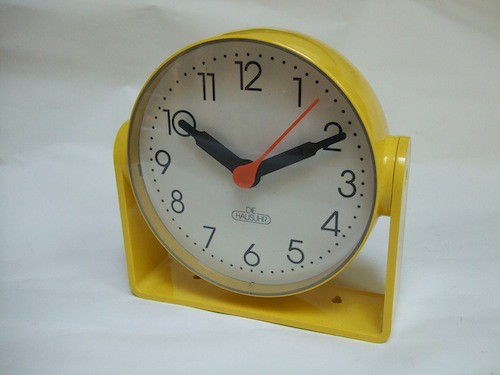In this image, a yellow-bordered clock with a built-in stand is prominently displayed on a white table or countertop. The clock features large, easy-to-read numerals and black hour and minute hands, with a red second hand providing a striking contrast. Just below the clock hands and above the 6 o'clock position, the brand name "Day Hauser" is elegantly printed. Additionally, the stand includes two small, circular openings, suggesting the option to secure the clock to a surface such as a table or bookcase.